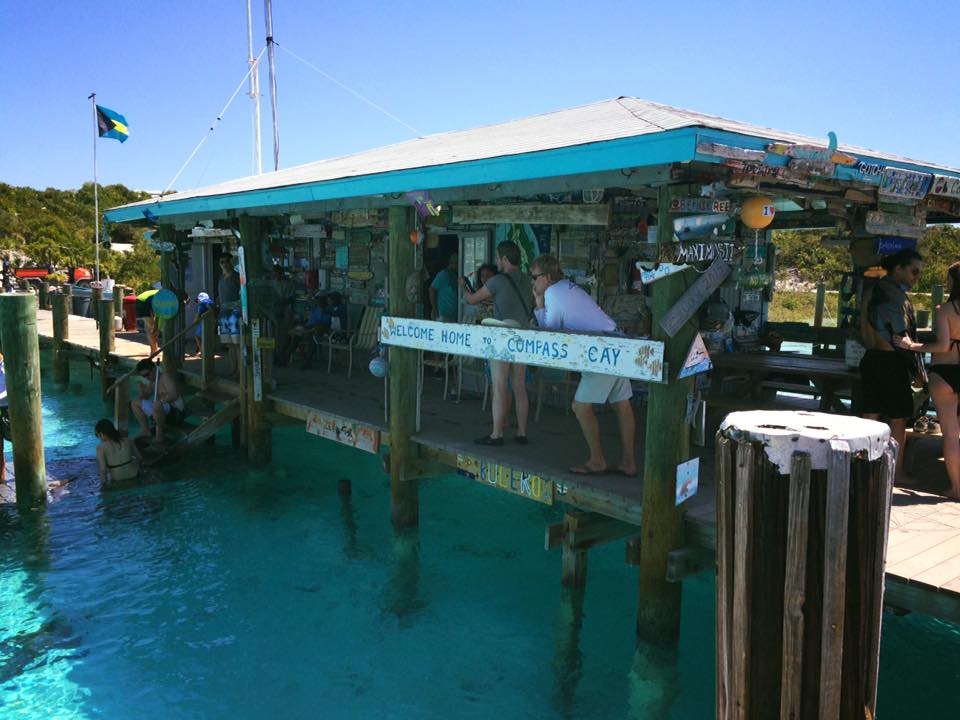This photograph captures a lively scene on a wooden pier extending over a clear, light blue tropical ocean. The sunny sky and distant green hills adorned with lush trees create a picturesque backdrop. The pier features a sheltered structure adorned with license plates and bumper stickers, possibly serving as a bar or a shop offering water sports equipment. At the center of the image, a mix of six people, including women in bikinis and men in swim trunks, are enjoying the sunny day. On the left side, a woman in a bikini stands on stairs leading into the water, half-submerged, while a man sits nearby. To the right, picnic tables and more people in swimwear are visible under the shelter. Prominently displayed on the right side is a white sign nailed to support beams, bearing the words "Welcome Home to Compass K" in blue text. A flagpole with a distinctive flag featuring yellow and blue stripes with a black triangle adds a touch of local charm to the scene. The image clearly depicts a bustling, inviting vacation destination.